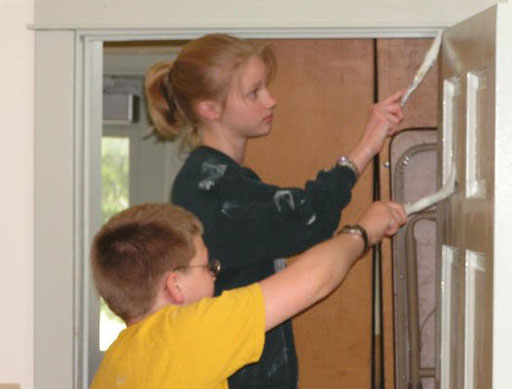In the photograph, an older sister and a younger boy are seen intently painting a doorway together. The older sister, positioned in the center of the doorway, has blonde hair tied in a ponytail and is dressed in a black top and a paint-splattered green sweater. She is focusing on painting the upper part of the open door and is wearing a watch on her painting hand. In front of her stands her younger brother, partially visible up to his armpits. He is sporting a close-cropped brownish-blonde haircut, glasses, and a yellow t-shirt, also adorned with a watch. They both hold paintbrushes coated in white paint, diligently applying it to the door’s interior. The backdrop reveals a room with light tan wooden walls and an exterior door with a window on the left side, allowing a view of the greenery outside.